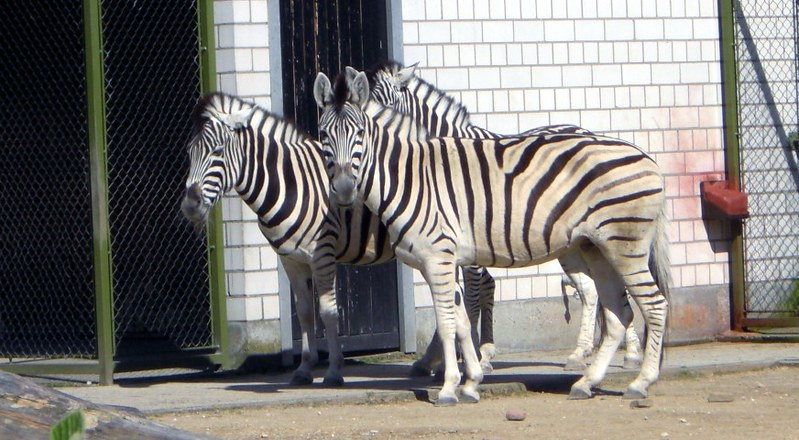This image captures three zebras standing in an enclosure at a zoo or animal park. The zebras, with their characteristic black and white stripes, are shown in profile against a white brick building. The enclosure is bordered by green chain-link fencing with green poles, adding a touch of color contrast. The ground beneath the zebras is a mix of concrete and dirt, scattered with round rocks. One zebra looks directly at the camera while the other two face straight ahead, offering a dynamic interaction with the viewer. Behind them, a red pipe extends from the wall, perhaps a water pipe used for animal care. Sunlight illuminates the scene, casting clear shadows and highlighting the zebras' unique stripe patterns. In the background, beyond the fence, there is a glimpse of green bushes, adding a touch of nature to the structured environment.